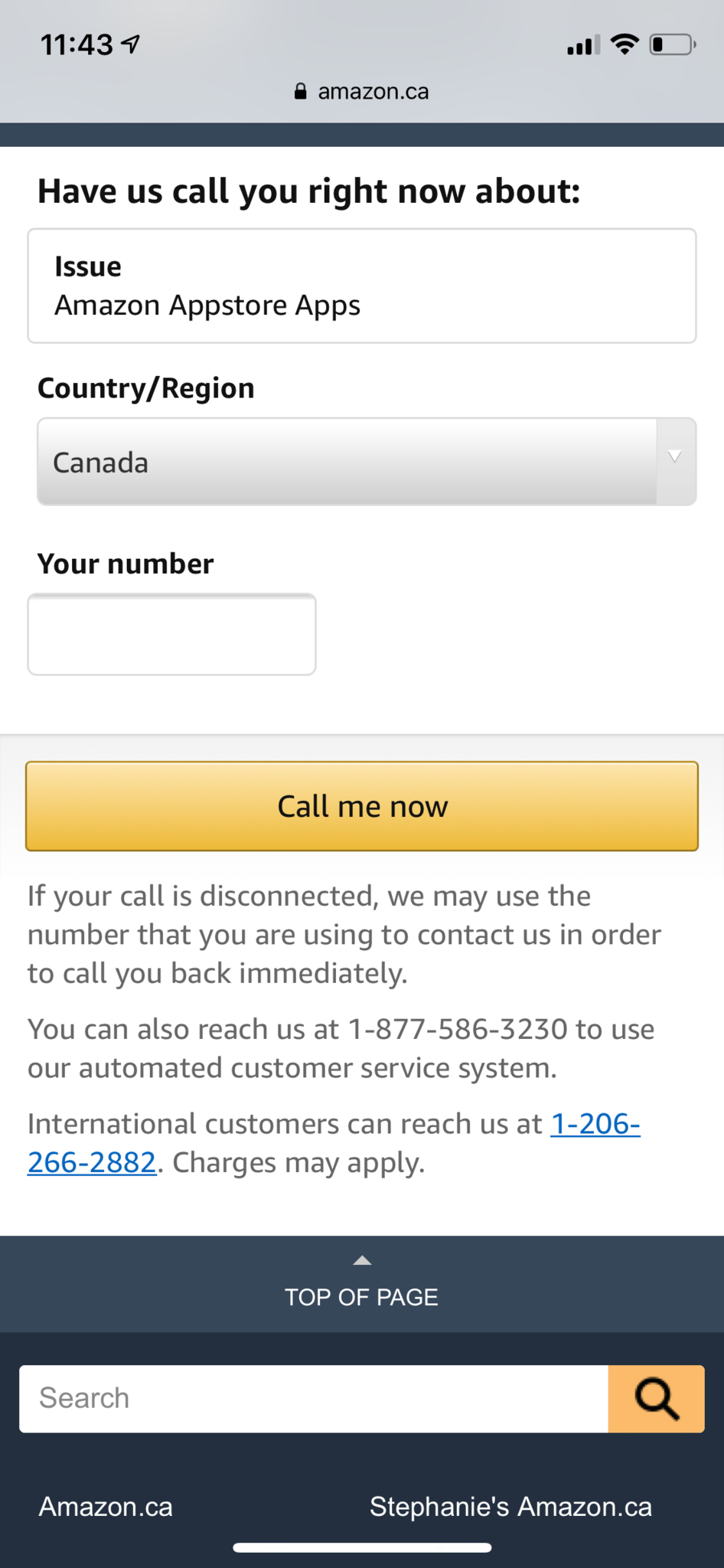This image, sourced from Amazon.ca, features a detailed customer service contact form for users in California. The layout begins with a light gray box at the top, followed by a darker gray box beneath it. The main section provides a prompt that reads, "Have us call you right now about," followed by a drop-down menu labeled "Issue," with "Amazon App Store apps" selected. Below, the form specifies "Country/Region" as "Canada" and includes a field labeled "Your Number" for users to input their phone number.

Further down, there's a prominent "Call me now" button. Below this button, there's a note: "If your call is disconnected, we may use the number that you are using to contact us in order to call you back immediately." A secondary contact option is also provided: "You can also reach us at 1-877-586-3230 to use our automated customer service system." For international customers, the form lists another number, "1-206-266-2882," with a disclaimer that charges may apply. At the very bottom of the image, there's a clickable link that allows users to return to the top of the page.